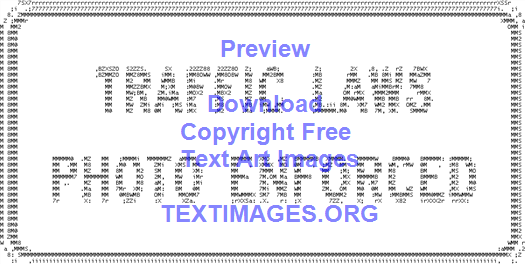The image depicts a rectangular design resembling a license plate with rounded corners. The rectangle has a pixelated border made up of small numbers and letters, giving it a distinctive digital texture. At the center, in blue lettering, are the words "Preview," "Download," "Copyright Free," "Text Art Images," and "TextImages.org," which are overlaid without regard to the underlying text, slightly obscuring it. The background features the words "Traffic Laws Photo Enforced" in a detailed, pixelated font composed of miniature numbers and letters. The overall color scheme is primarily black and white, with the blue text standing out prominently. The design seems to be a clip art template suitable for various projects.